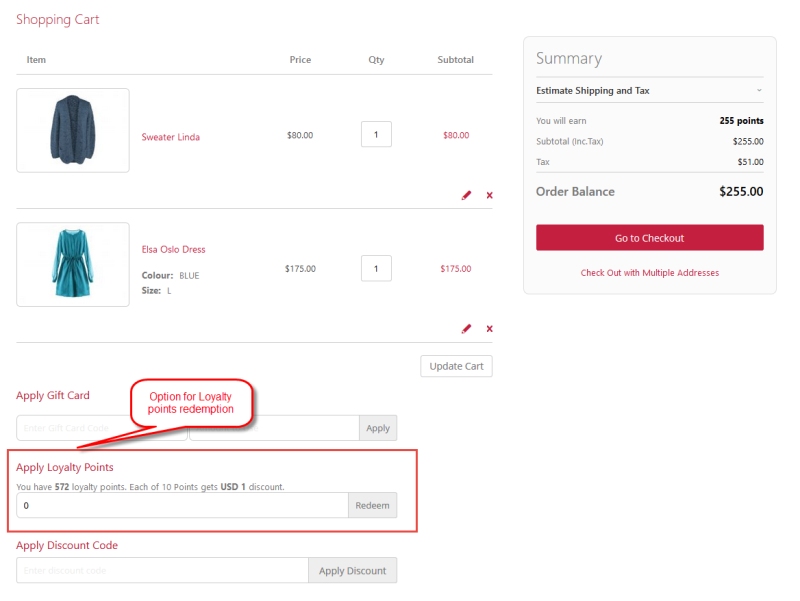**Screenshot Description: Online Shopping Cart Overview**

This screenshot captures a user's online shopping cart on a retail website. In the top left corner, a bold red label reads "Shopping Cart." Below this heading, the main content is divided into sections:

- **Product List**: The upper section prominently features item thumbnails with descriptions:
  - Top-left: An image of a suit jacket.
  - Below: An image of a blue dress labeled as "Sweater Linda."
  
  Each product listing includes details like the name, price, quantity, and subtotal. There are options to edit or remove items from the cart.

- **Discounts and Rewards**: Beneath the product list, there are fields for applying discounts:
  - **Gift Card**: A white rectangle to enter the code.
  - **Loyalty Points**: Highlighted by a large red rectangle with a note in a red speech bubble, mentioning "option for loyalty points redemption."
  - **Discount Code**: Another field for discount codes.

Each field has a corresponding "Apply" or "Redeem" button to the right.

- **Order Summary**: Positioned in the top right, a summary box includes:
  - Estimated shipping and taxes.
  - Points earned through this purchase.
  - Subtotal, tax, and the final order balance.
  
  Below the summary, a prominent red button labeled "Go to Checkout" is displayed, with a smaller button beneath it for the option to "Checkout with Multiple Addresses."

This detailed view provides a comprehensive look at the user's shopping cart, emphasizing discounts and the total order cost.